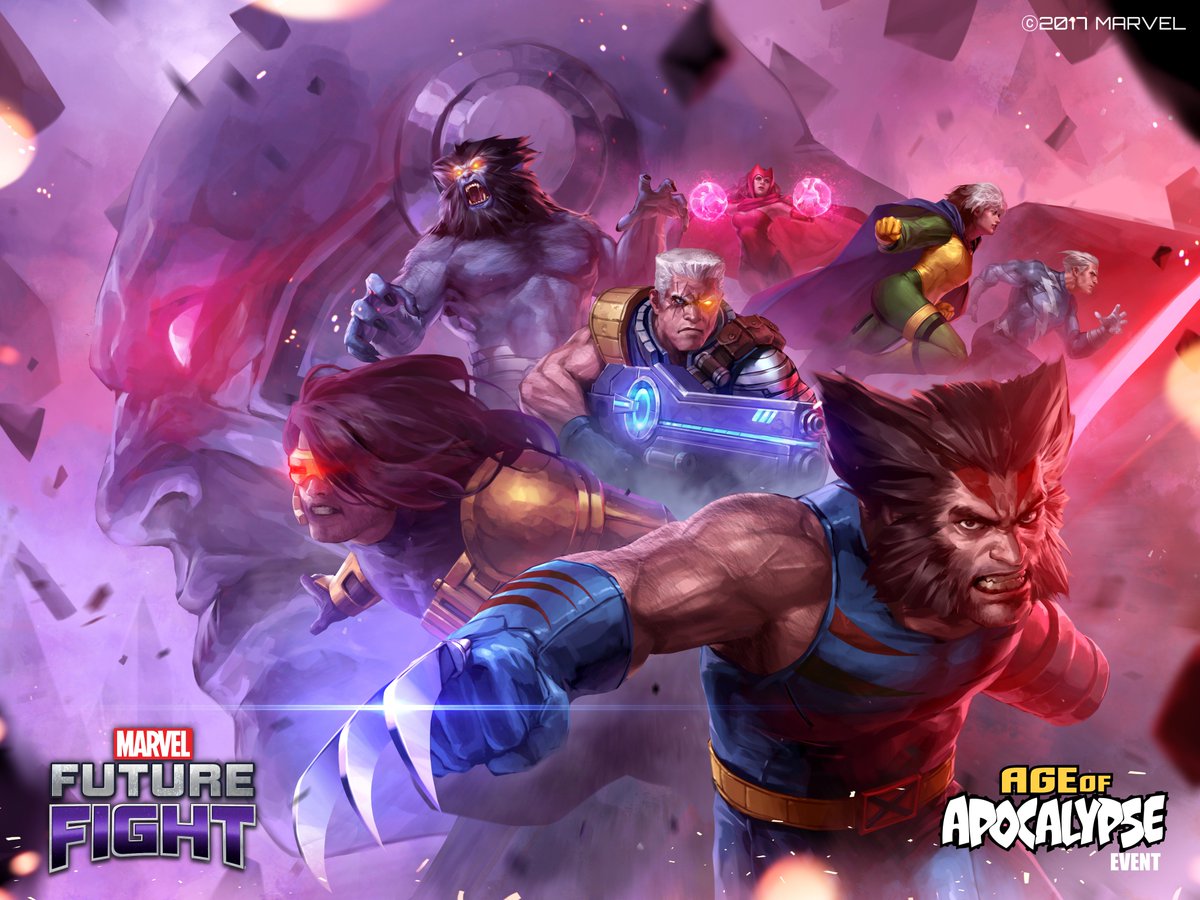This dynamic advertisement for the video game "Marvel Future Fight" exudes a captivating space-themed aesthetic. Dominating the background is a visually striking figure with a purple hue, a bald head adorned with menacing spikes, and a mysterious circular device over their ear. Their intense, glowing red eyes gaze to the left, adding an element of intrigue and foreboding.

In the forefront, an ensemble of superhero-like characters demands attention. A menacing werewolf-like figure, distinguished by luminescent yellow eyes and razor-sharp claws, appears ready for action. Adjacent to this character stands a female figure, her red complexion accentuated by the radiant pink orbs she wields in her hands. Adding to the diverse roster, a man with stark white hair and a single yellow eye stands clad in a military uniform, confidently holding a large blue gun.

On the bottom right, a character resembling Wolverine commands the scene with his iconic brown hair, blue gloves, and razor-sharp claws. He is outfitted in a blue shirt with a distinctive yellow band. Positioned behind him, a female character with brown hair and glowing red eyes adds to the formidable team assemblage.

Prominently displayed in the bottom left corner is the unmistakable red logo of "Marvel Future Fight." In the bottom right corner, the text heralds an exciting "Age of Apocalypse Event," with "Age of" in bold yellow lettering and "Apocalypse Event" in striking white.